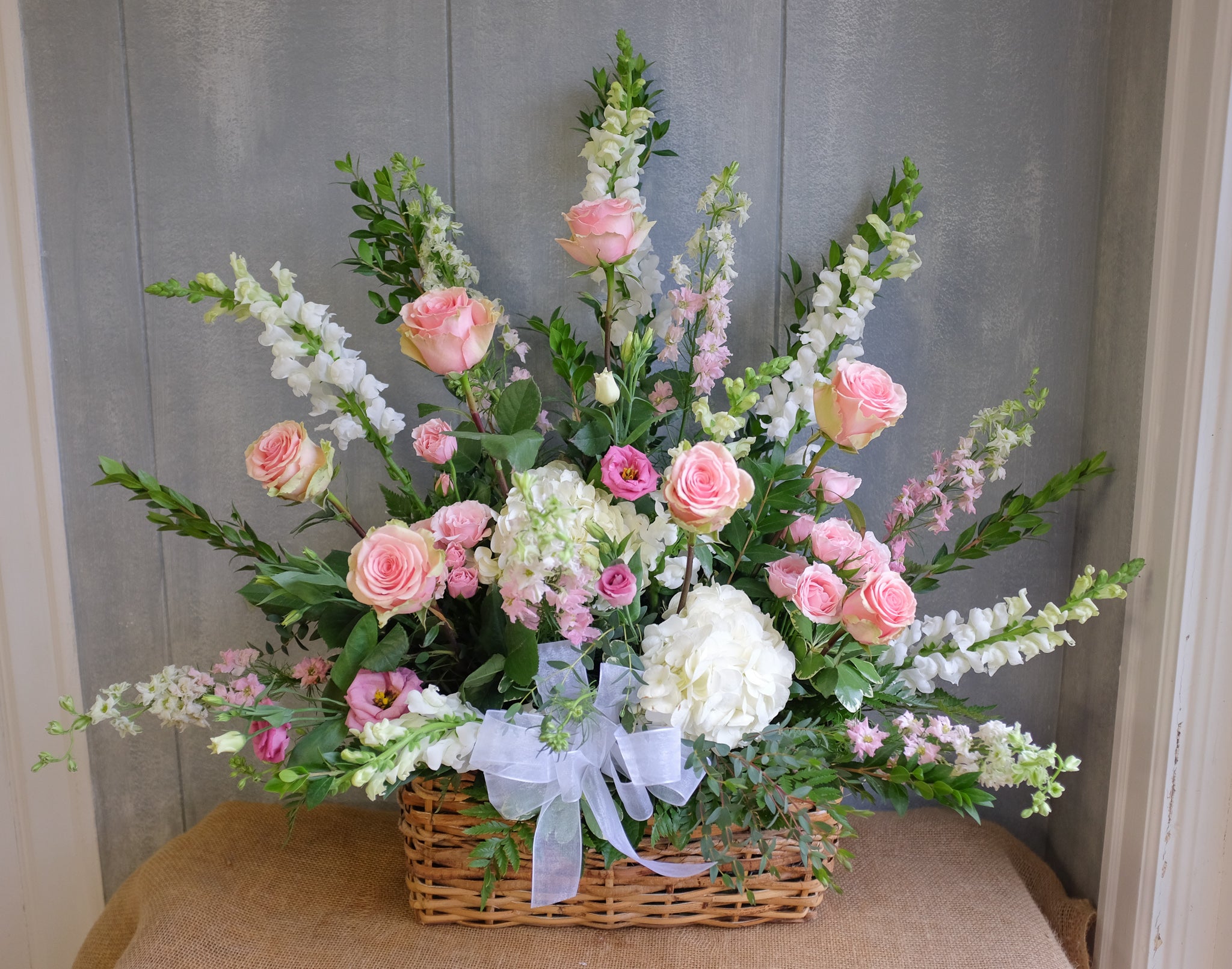This color photograph, oriented in landscape, captures a detailed scene centered around a flower arrangement. The vibrant bouquet is nestled within a light brown wicker basket, which itself is positioned on a table draped with a brown tablecloth. The rustic wicker, interwoven with straw pieces, gives the arrangement a charming, natural touch. A light purple silk bow, tied with multiple loops, accents the top of the basket.

The bouquet is lush with green stems and leaves fanning out in various directions. The centerpiece features large white flowers, likely white hydrangeas and snapdragons, accompanied by light pink and blush roses, creating a delicate color contrast. The arrangement also includes sprays of white hollyhock flowers, their elliptical shapes adding to the radial symmetry of the display.

Behind the arrangement is a backdrop of gray-washed vertical panels, streaked with white and divided by thin black lines. These panels are framed on both sides by what appears to be parts of a white-painted window frame, adding a quaint architectural element to the composition. The scene is skillfully composed, blending natural elements with a subtle background, highlighting the vibrant florals as the focal point.